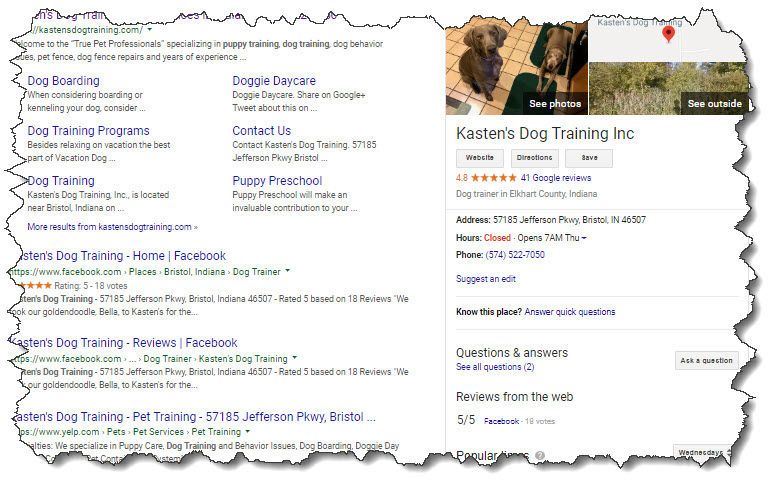An image displays a torn fragment resembling a Google search result, creating the appearance that the edges have been ruggedly shredded. The rectangular shape, which is longer horizontally, gives the impression of accidental damage, yet cleverly ties into the theme of the search.

The search query appears to be related to dog training, highlighting a somewhat ironic twist given the tattered state of the image. The focal point is "Kaiser's Dog and Training Incorporated," a dog training service with a 4.8-star rating based on 41 Google reviews. Details provided include:

- **Location:** Dog trainer in Ecknard County, Indiana
- **Address:** 57185 Jefferson Parkway, Bristol, Indiana 46507
- **Hours:** Closed at the time of the query, with a note of opening at 7 a.m. on Thursday
- **Phone:** 574-522-7050

The image also suggests functionality for edits and quick answers, showing snippets of reviews from the web, including a perfect 5 out of 5 rating on Facebook from 18 votes.

The visual metaphor is both whimsical and clever, making it appear as though a mischievous dog shredded a Google search page, driving home the point that dog training might be a necessary next step for the pet owner.